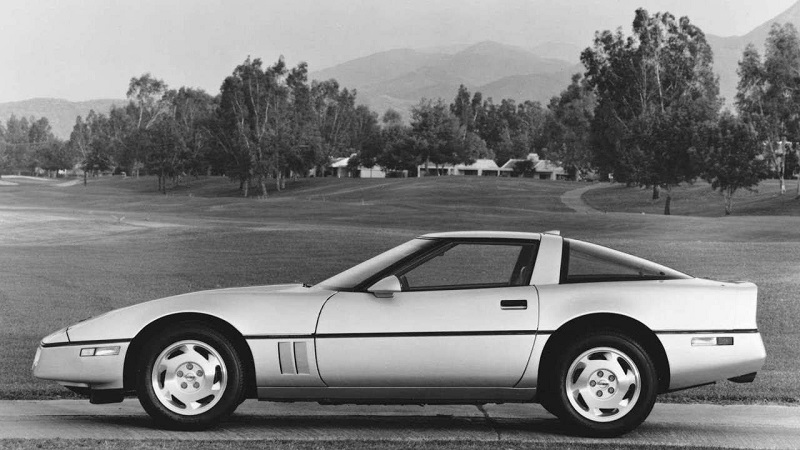This black-and-white photograph captures a side profile of what appears to be a 1980s-style Corvette, potentially a Chevrolet Corvette, parked on a narrow cement road in a rural setting that resembles a golf course. The sleek, light-colored sports car, possibly white or silver, shows off its unblemished, shiny surface, with clean, reflective windows and wheels. The car is oriented with its headlights to the left and rear to the right. Surrounding the car is a lush landscape characterized by expansive grassy areas, scattered mature trees, and gently rolling hills in the background. A white building, reminiscent of a golf clubhouse, is situated amidst the trees, with one-story homes outlining the scene. In the furthest distance, high mountains rise above the tranquil rural panorama.